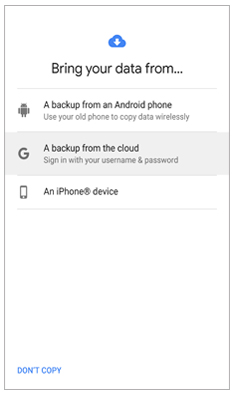This screenshot captures a cloud syncing interface on a mobile phone, designed to help users transfer their data. 

The background is white, giving a clean, minimalist appearance. At the top center, there is a prominent blue cloud icon with a white downward-pointing arrow at its center, symbolizing data download or syncing.

Below the cloud icon, the interface reads "Bring your data from," in large, bold black letters, making it clear what the screen is instructing.

Three options are listed vertically for data transfer:

1. The first option displays an Android icon on the left, followed by the text "A backup from an Android phone," in bold black font. Beneath this, it instructs users to "Use your old phone to copy data wirelessly," providing guidance on the process.
   
2. The second option features a Google logo on the left and the text "A backup from the cloud," in bold black writing to the right. Below this, it advises users to "Sign in with your username and password" in smaller gray letters, indicating the need for a Google account login.

3. The third option shows an iPhone icon on the left with the text "An iPhone device" to its right, suggesting compatibility with Apple devices for data transfer.

At the bottom left corner of the screen, there is an option labeled “Don’t copy” in small blue capital letters, offering users the choice to bypass the data transfer process.

The rest of the image appears to be cropped, focusing attention on these key elements.